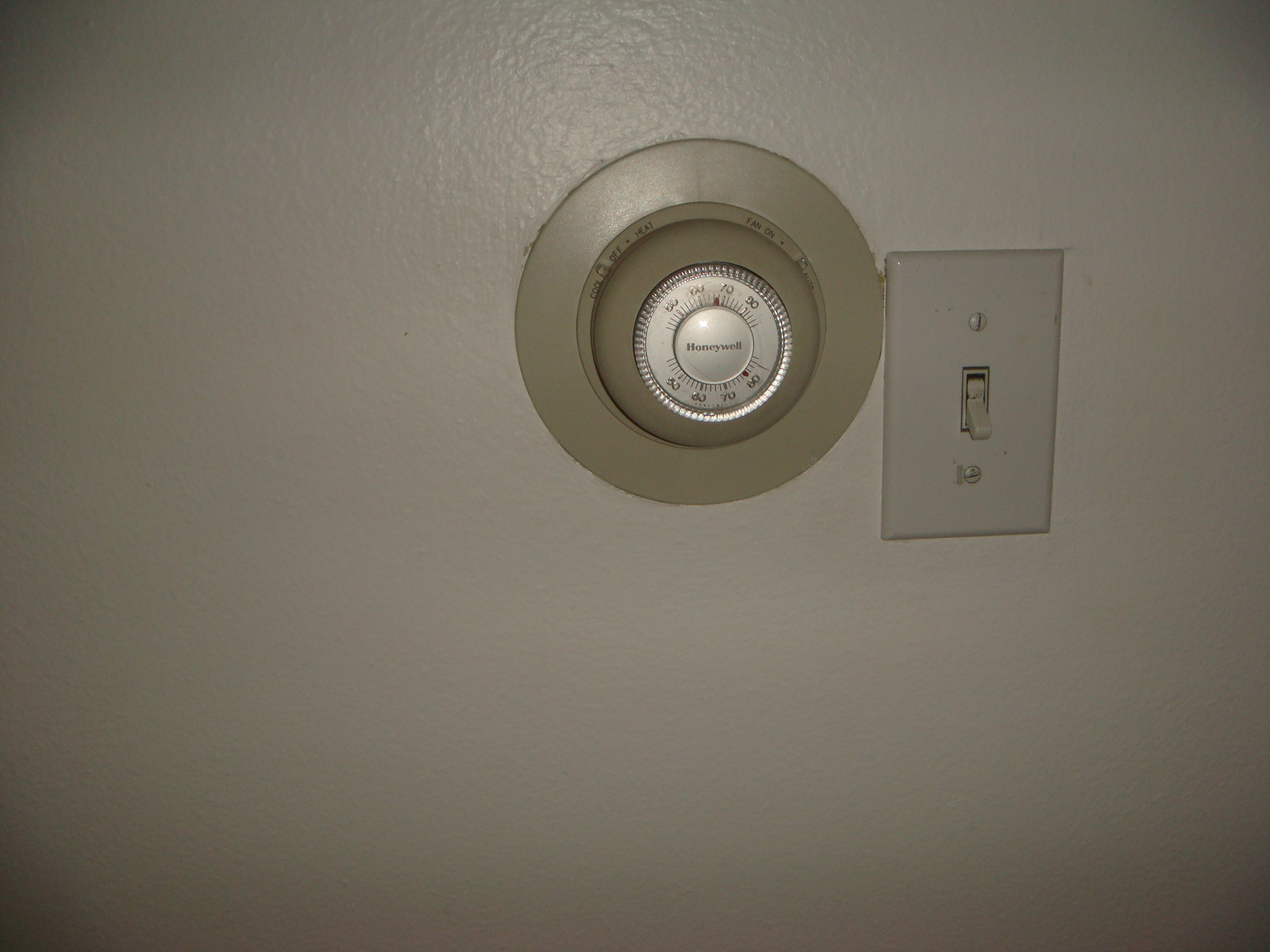This photograph features a vintage Honeywell thermostat mounted on a clean, white wall, likely dating back to the 1970s or 1980s. The thermostat is positioned in the upper middle section of the frame and is adjacent to a single light switch on its right, with the switch currently in the down position. The thermostat itself is a classic circular model with a beige outer ring and a silver central area where the brand name "Honeywell" is prominently displayed in black text. Surrounding the brand name are temperature markers, with numbers ranging from 50 to 80, repeated on both the top and bottom hemispheres. The device has an array of settings labeled on its surface: the upper left quadrant indicates "cool," "off," and "heat," with a small lever between "cool" and "off," while the upper right quadrant shows "fan on," accompanied by another small stopper. The nostalgic design and tactile controls of the thermostat make it a notable relic from a bygone era, contrasting with the simplicity of the modern light switch beside it.